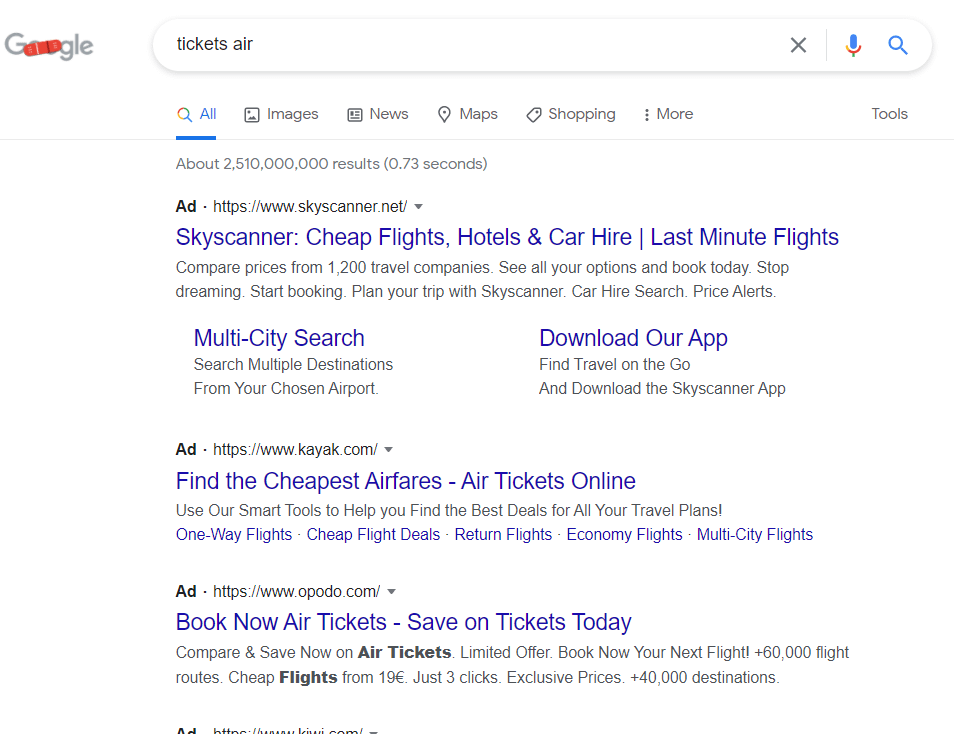Screenshot of a Google search results page:

In this screenshot, the Google logo in the upper left-hand corner, typically adorned in vibrant rainbow colors, is displayed in gray with a band-aid covering the two O's. This unique logo alteration suggests a themed presentation, possibly referencing a temporary issue or problem. The search query entered is "tickets air," and a microphone icon indicates the use of a voice command for input.

Beneath the logo, the search options bar offers various categories to refine the search results: All, Images, News, Maps, Shopping, and More, with additional tool options situated on the far right. An impressive approximate count of 2,510,000 results is displayed, achieved in a swift 0.73 seconds.

The search results are highlighted by three advertisements:
1. The first ad from Skyscanner.net promotes cheap flights, hotels, and car hires, alongside options for last-minute flights, multi-city searches, and a prompt to download their app.
2. The second ad from Kayak.com emphasizes finding the cheapest airline tickets online, curiously noting the unrelated name association.
3. The third ad from Opodo.com encourages users to book tickets now to save on fares today.

The background remains Google's signature white, with the ad text in black, and the websites in black as well. The hyperlinks stand out in the familiar light-ish dark blue, characteristic of Google's typical design. The page is concise, showcasing only these three ads related to the search query.